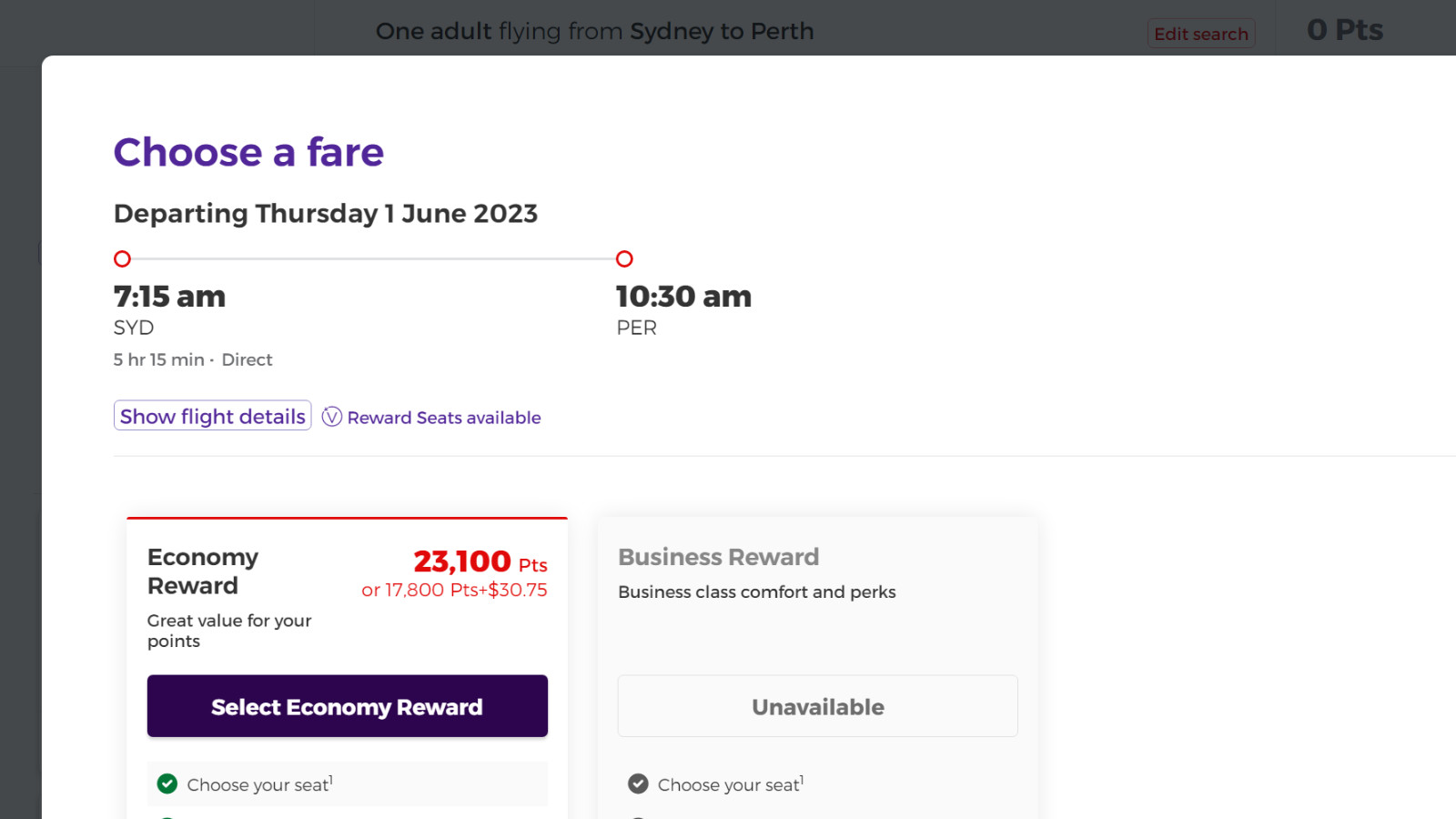A detailed view of a flight booking website interface. In the background, the top and left sections are occupied by a semi-transparent, faded light black overlay. This section indicates travel details: "One adult flying from Sydney to Perth." The top right displays options: "Edit," "Search," and "0 points."

Dominating the image, the foreground features a prominent white pop-up window that covers most of the screen. At the top left of the pop-up, the heading "Choose a fare" in purple is visible. Below this, the departure details are outlined: "Departing Thursday, 1st June 2023, 7:15 AM, Sydney," followed by "5 hours, 15 minutes direct" and an arrow pointing to "10:30 AM PER (Perth)." Below this, the options "Show flight details" and "Reward seats available" appear in purple text.

At the bottom left corner of the pop-up, a white rectangle provides economy fare options. It starts with "Economy Award: 23,100 points or 17,800 points + $30.75," and a subtext, "Great value for your points." A prominent purple button with white text reads, "Select Economy Reward," accompanied by a green checkmark that signifies "Choose your seat."

On the right side, a faded gray rectangle shows details for business class. The text "Business Reward" is followed by "Business class comforts and perks," but this option is marked as "Unavailable" within a gray-bordered button.